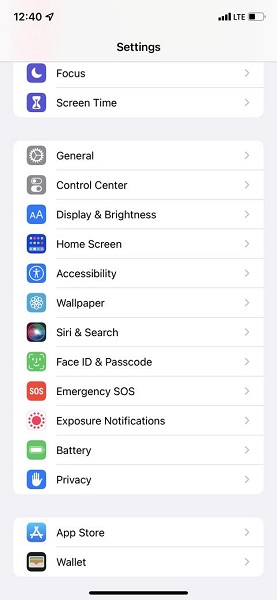This screenshot depicts the settings menu of a device. At the top, there are two primary tabs labeled "Focus" and "Screen Time." Below these tabs, within a large rectangular section, there is a comprehensive list of various settings options, each accompanied by a distinctive icon to its left. This list includes more than ten different tabs: General, Control Center, Display & Brightness, Home Screen, Accessibility, Wallpaper, Siri & Search, Face ID & Passcode, Emergency SOS, Exposure Notifications, Battery, and Privacy.

Each icon is a colored square with a unique symbol; for instance, the Privacy tab is marked with a blue square featuring a white open palm. At the very bottom of the settings menu, separated within a white rectangular section, are two additional options: App Store and Wallet. The organized layout and vivid icons make navigation user-friendly and efficient.